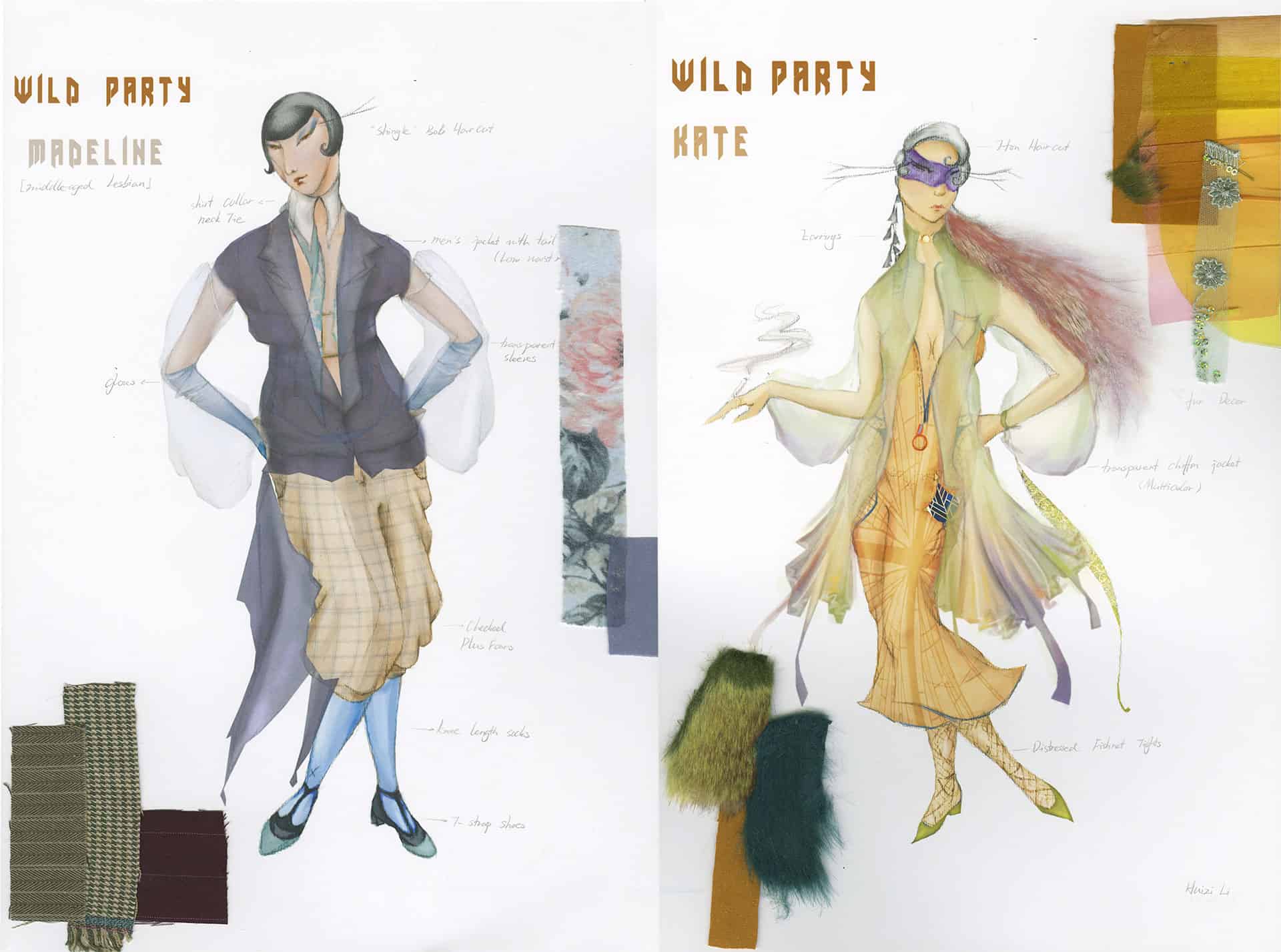In this visually striking illustration, we see side-by-side fashion designs labeled with brown text at the top: "Wild Party." The left image is titled "Madeline" and the right "Kate," as noted in contrasting grey and orange hues respectively. 

Madeline, depicted on the left, embodies a quirky, playful style with her short, sleek black hair and banged eyebrows. She wears a collared shirt paired with a short-sleeve, black cropped jacket with flowing coattails. Blue elbow-high gloves add a splash of color, complementing her loose-fitting plaid pants that fall just below the knee, along with blue socks and green-and-black shoes. Her look is accentuated by her confident pose, with hands firmly placed on her hips.

To the right, Kate exudes a more sophisticated flair. She sports gray hair and a purple eye mask, alongside long earrings and a red feathery accessory that elegantly drapes from her head to her arm. Her attire includes a semi-transparent, greenish overcoat with a gradient blend of purple and orange at the hem, and loose, flowy sleeves. Beneath this overcoat, Kate wears a gold dress adorned with geometric prints. Her ensemble is completed by lacy stockings and green high heels. In her poised demeanor, she holds a cigarette in one hand while resting her other hand on her hip.

Both illustrations are detailed with additional textile samples glued at the corners, adding a tactile dimension to the artwork. The contrast in their outfits—Madeline's avant-garde, vibrant look versus Kate's opulent, flowing elegance—creates a captivating juxtaposition, highlighting diverse facets of fashion illustration.